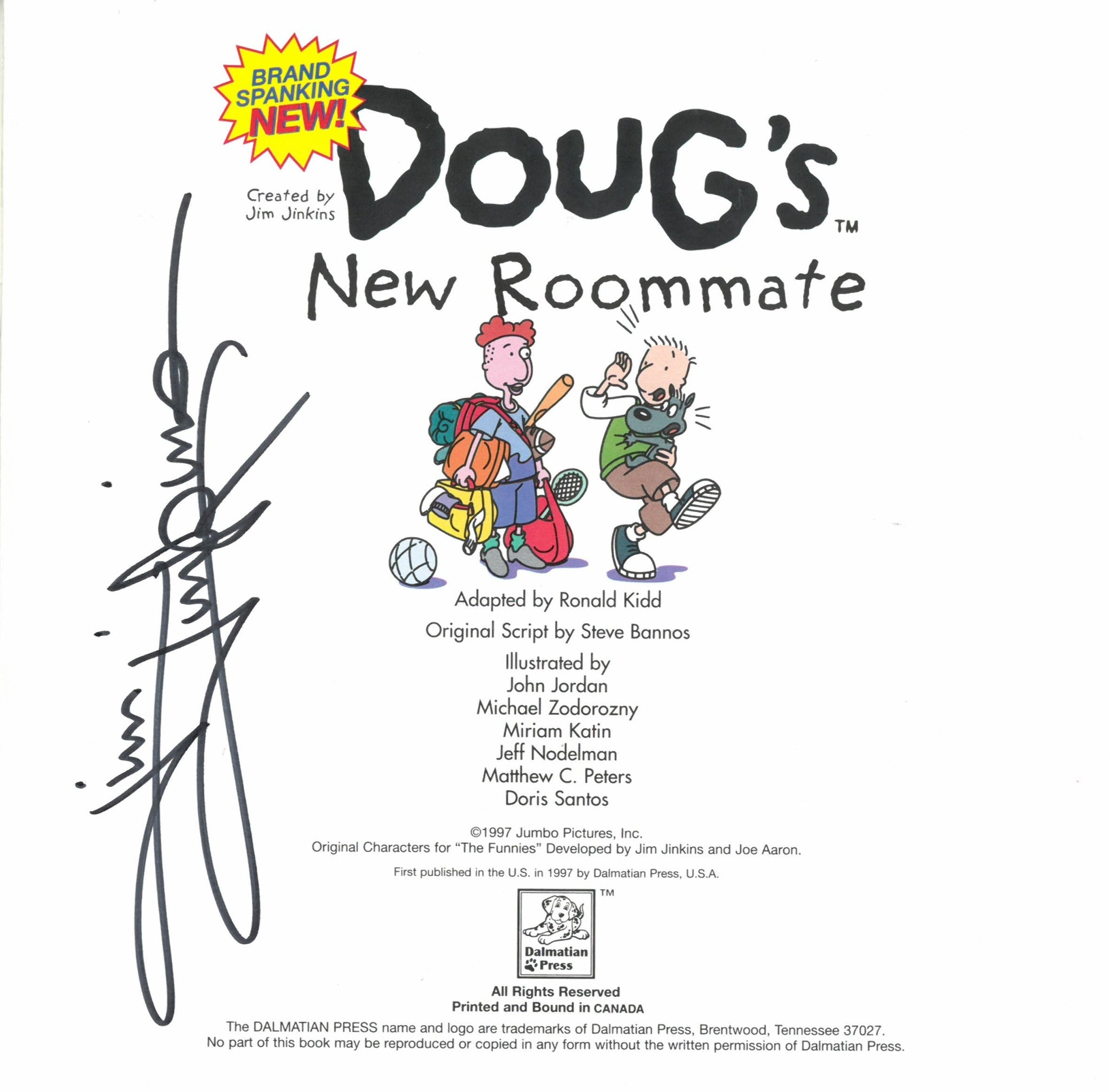This is an inside front cover for the book titled "Doug's New Roommate." In the upper left-hand corner, there is a prominent yellow starburst design outlined in red, reminiscent of an explosion, with the text "Brand Spanking New" in black letters. The title "Doug's New Roommate" is written in very large letters with a trademark symbol next to "Doug's," and beneath that, it states "Created by Jim Jenkins" in black writing. Jim Jenkins' signature runs vertically along the left-hand side of the page.

Centered on the page are two cartoon figures, both male. The first figure, depicted in a pink hue with red hair, is loaded with numerous multicolored objects including yellow, orange, and red bags, as well as various sports equipment: a football, a baseball bat, a tennis racket, and a sleeping bag on his back. A soccer ball appears to be at his feet. The second figure, in peach tones, is portrayed walking forward with one foot raised as if in motion, holding a startled dog. He is dressed in brown pants, a green top, and a white button-down shirt underneath.

The page also contains detailed credits and copyright information at the bottom, reading: "Adapted by Ronald Kidd, Original Script by Stephen Banos, Illustrated by John Jordan, Michael Zoder-Rosney, Marian Caton, Jeff Nodelman, Matthew C. Peters, Doris Santos, 1997, Jumbo Pictures."